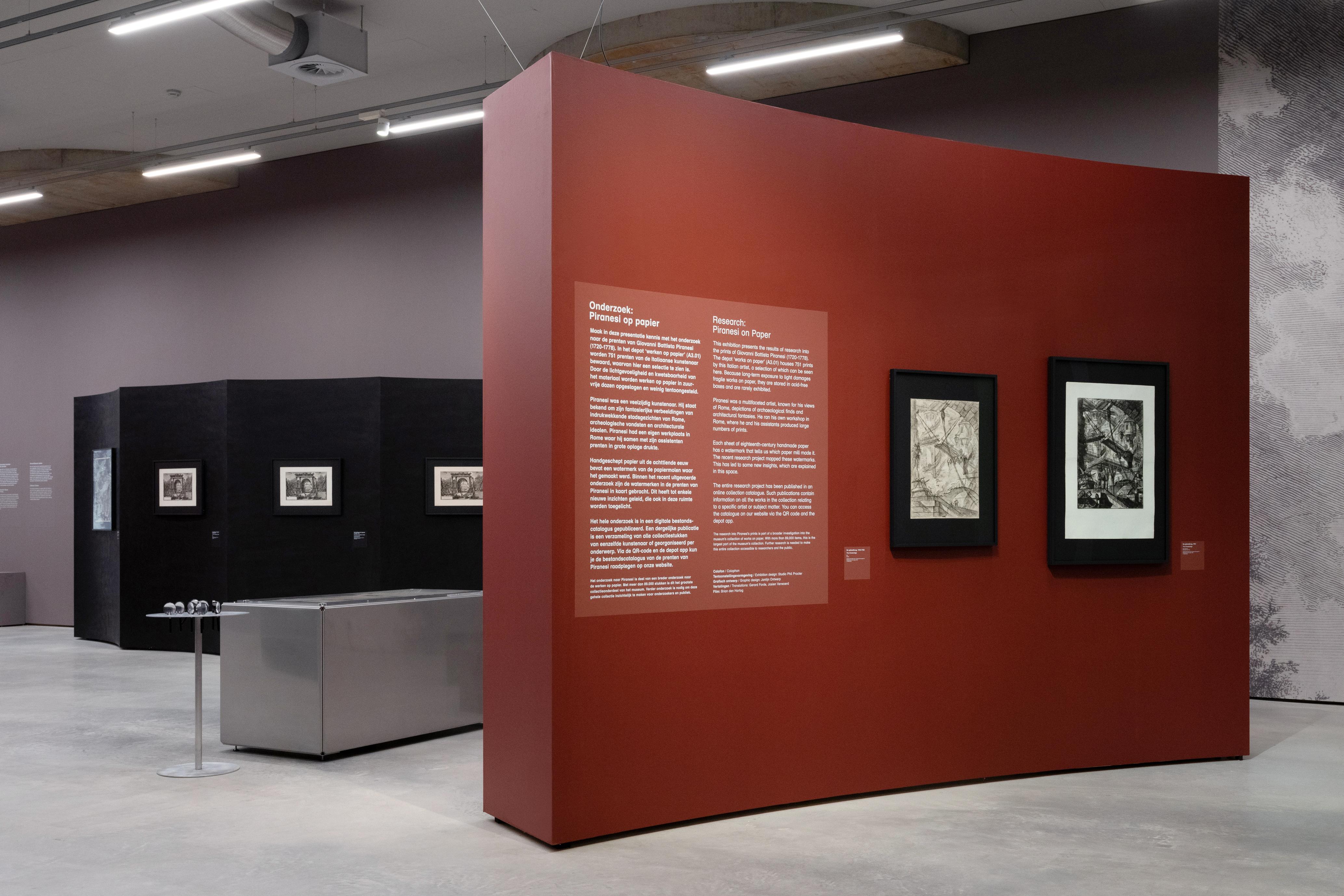The image depicts an art gallery with an industrial ambiance accentuated by concrete floors and walls. Central to the photograph are two low display walls—one black and one maroon red. The red wall, situated in the foreground, prominently features a large panel with two columns of white text, likely providing information about the artist or the artwork. Affixed to this red wall are a few black-and-white artworks in black frames, creating a stark contrast against the maroon background. In the middle of the space, perhaps serving as a focal piece, is a sleek silver cabinet, which could be interpreted as a table or bench. Further into the background and to the left, the black display wall exhibits three pieces of black-and-white artwork, each uniquely framed and part of a cohesive series. Overhead, the gallery is illuminated by multiple fluorescent lights hanging from rails, casting a clear light on the artworks and enhancing the clean, industrial aesthetic of the space.